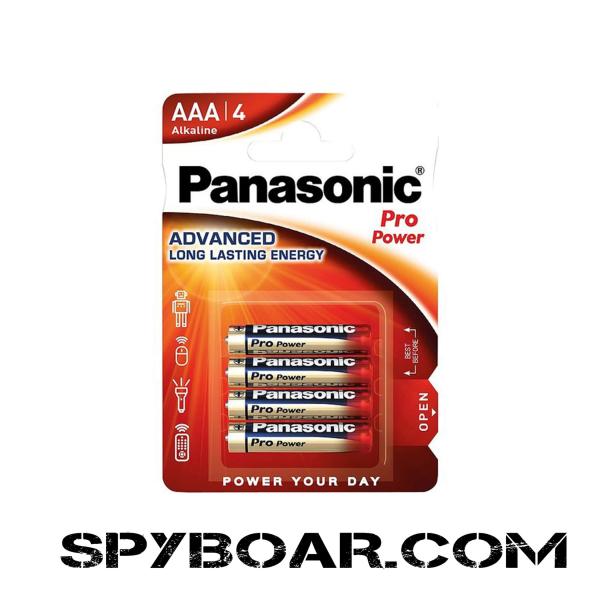The image features a blister pack of Panasonic AAA batteries, showcasing four batteries aligned vertically. The packaging prominently displays the brand "Panasonic" and identifies the batteries as "Pro Power" with the phrase "Advanced Long-Lasting Technology" highlighted in blue text below. Above these descriptions, the number "4" next to "Alkalon" is visible, indicating the pack size. 

The packaging also includes visual icons representing a robot, a mouse, a flashlight, and a remote control, suggesting the types of devices the batteries are suitable for. The phrase "Power Your Day" is prominently displayed, emphasizing the batteries' reliability for everyday usage. An indentation in the form of two triangles, with their tips pointing towards each other, is located on the right side of the packaging. In the space between the triangles, there is a pull tab, signifying an easy-open feature. Additionally, the website "spyboar.com" is mentioned on the packaging, though it appears slightly ambiguous due to the way it is printed.

Each individual battery is branded with "Panasonic Pro Power" to maintain consistency with the packaging's theme.